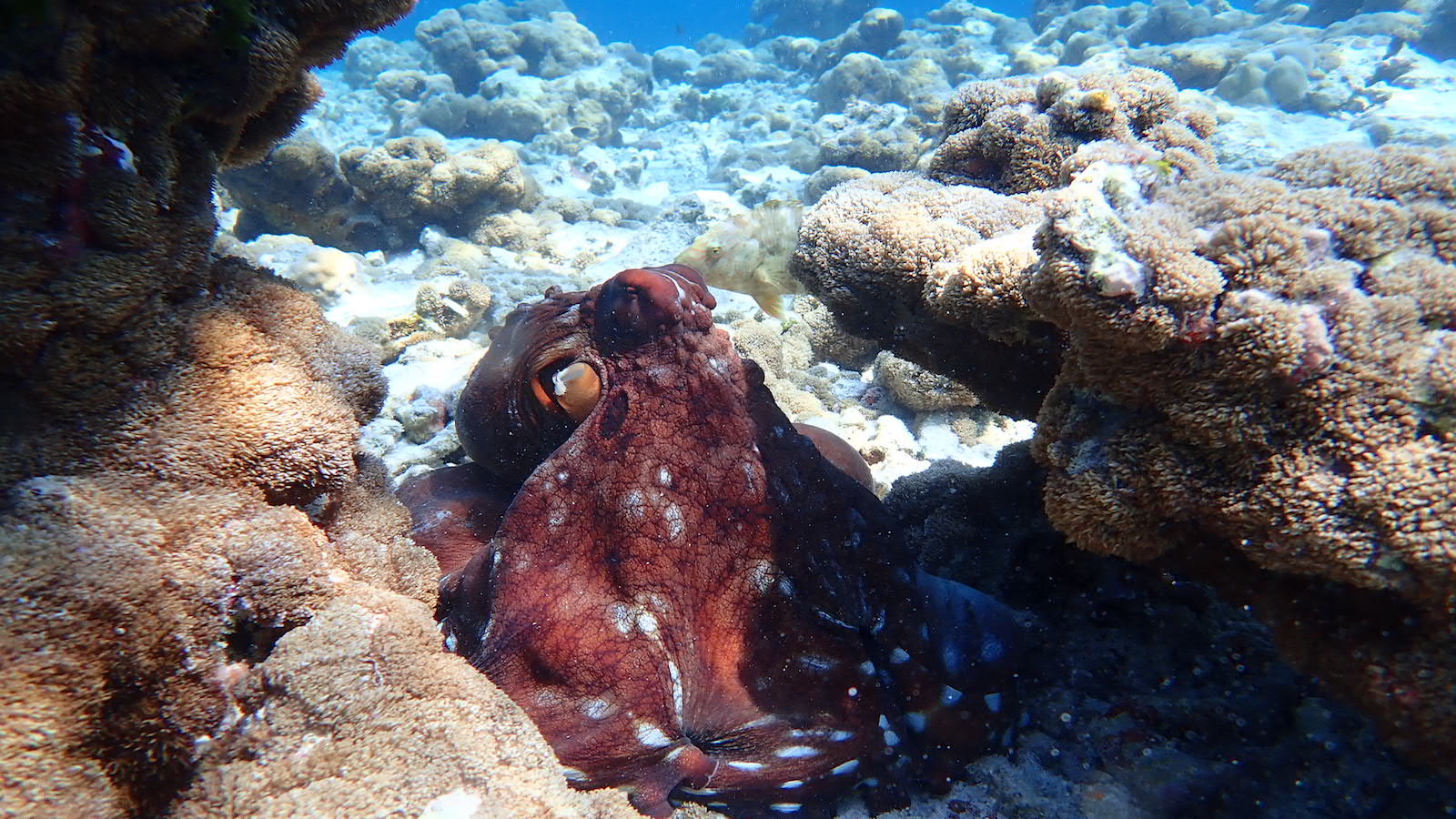This underwater photograph features a dark red octopus with white and grayish spots, positioned centrally amidst an array of coral reefs. The octopus, appearing sleepy and dormant, is viewed slightly from behind, showing its left eye. Surrounding the octopus are stacks of tan coral reefs, with the left stack extending vertically from the bottom to the top of the image, and the right stack rising almost to the top, jutting inward. The background is predominantly blue, featuring additional beige coral, white rocks, and particles resembling dust scattered around, especially in the bottom right. Light rays penetrate the water from the top of the image, creating a mystical underwater ambiance. Notably, there is also a brown fish partially hidden behind the coral on the right side of the frame. The overall image has a blurry quality, similar to that of a photograph of a photograph.